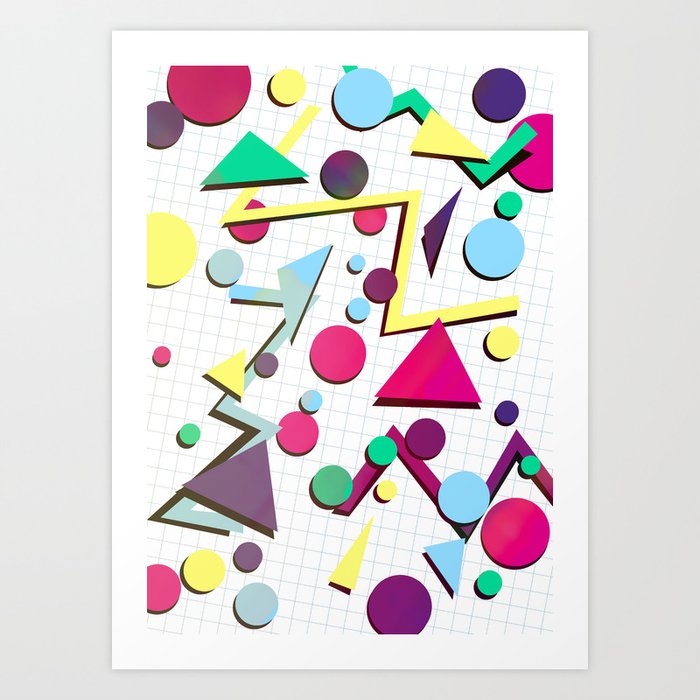The image is a photograph of a vertically aligned, modern art style poster placed on a grayish surface. The poster features a white background overlaid with a light gray, slightly tilted diagonal grid resembling graph paper. Atop this grid, there are various computer-generated geometric shapes in bright colors, including pink, yellow, blue, green, and purple. The shapes, which include circles, triangles, and zigzag lightning bolts, appear to be of different sizes and are randomly arranged, often overlapping each other. Notably, the largest circle is pink, the largest triangles are pink and purple, and the largest zigzag is yellow. Additionally, there are light blue and darker blue zigzags and triangles. Each shape casts a narrow dark shadow to the bottom left, suggesting a light source from the upper right. The arrangement and vividness make it a funky, colorful piece of geometric artwork.